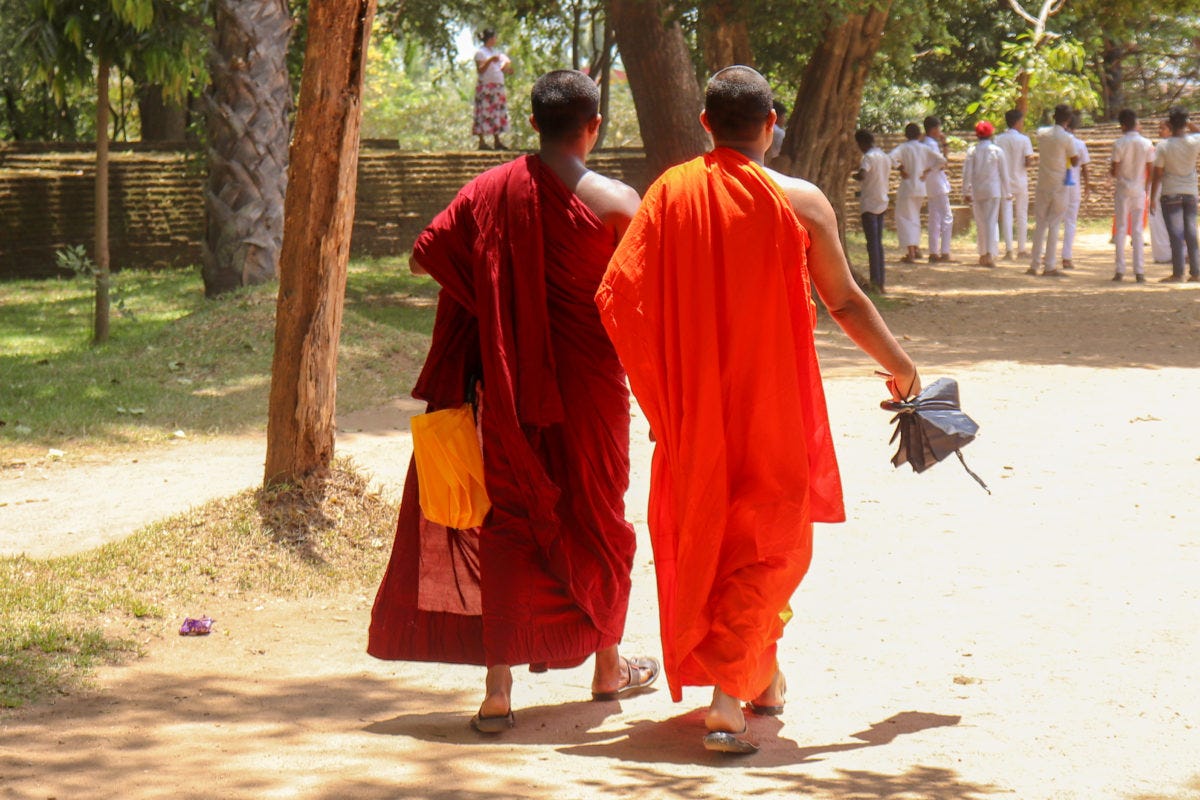The image captures the back view of two Buddhist monks walking along a dirt path toward a serene garden setting. On the left, the monk is dressed in a deep red robe, with his right shoulder exposed, and he holds an orange umbrella in his left hand. The monk on the right wears a bright orange robe, similarly exposing his right shoulder, while holding a black umbrella in his right hand. Both monks are wearing sandals. To their left, several tree trunks and perhaps a fence are visible, creating a natural border to the scene.

Ahead of the monks, a group of people, mostly dressed in white, can be seen, some wearing jeans and white t-shirts, while others are clad in more traditional white outfits. They all stand with their backs to the camera, facing a wall that borders a lush area filled with trees. Among the group, occasional turbans are visible, adding to the cultural richness of the scene. The mix of natural elements, traditional attire, and the group of people suggests that a significant ceremony or event may be about to take place.